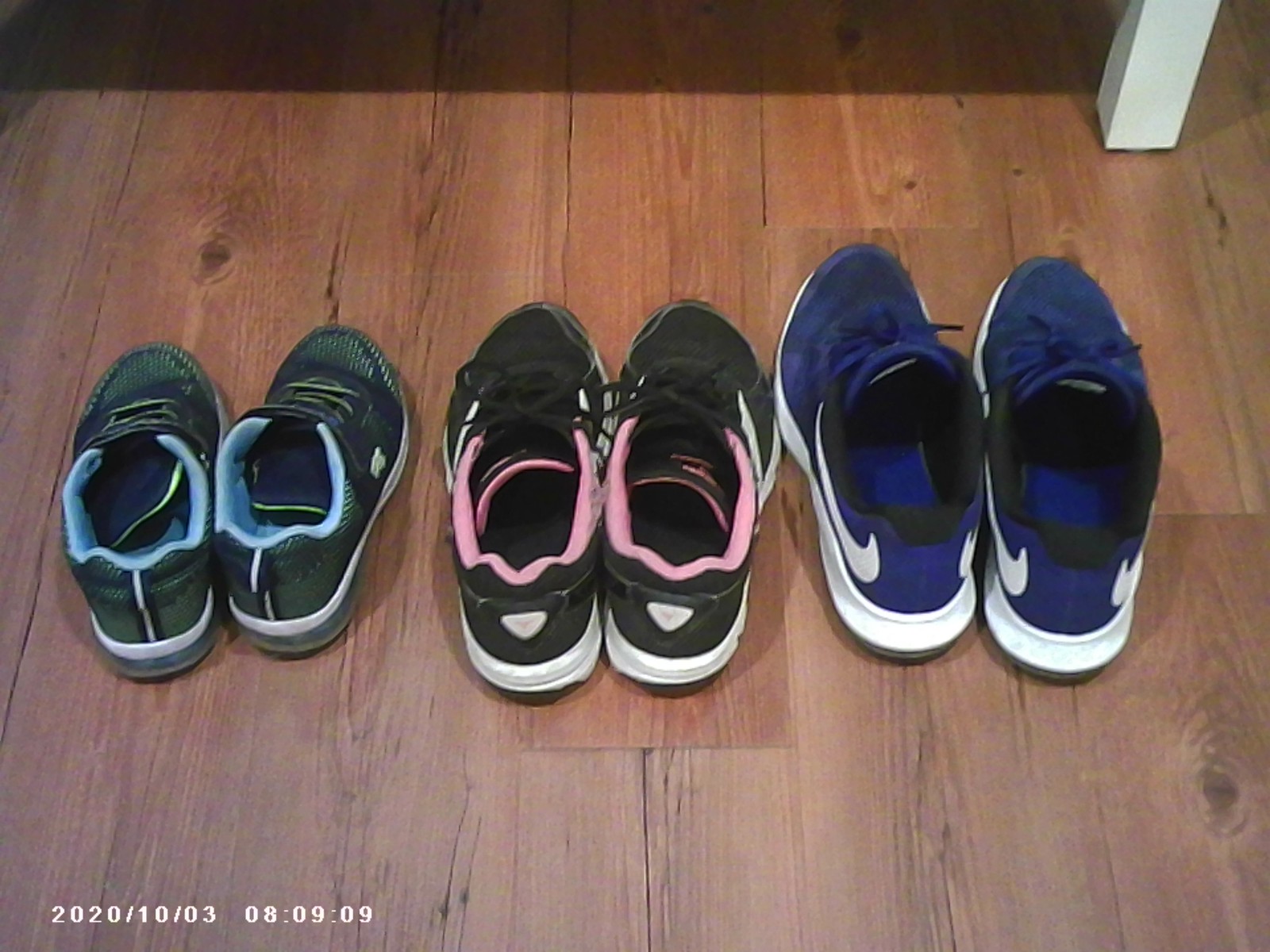This image depicts three pairs of children's trainers neatly aligned on a brown wooden floor. The floor's hue transitions from darker at the top to lighter towards the bottom, a likely effect of the lighting. In the lower left corner, a digital watermark displays the date "2020-10-03" and the time "08:09:09." The upper right of the photograph features a rectangular white table leg or structural element.

From left to right, the shoes increase in size. The leftmost pair is primarily dark green with blue highlights, including light blue on the inside, and white accents on the back and soles. The middle pair appears dark green, with pink on the top and tongue and white highlights, including white triangles at the back. The rightmost pair is predominantly dark blue with black accents around the ankle area, a white Nike swoosh on the sides, and white detailing on the soles.

The trainers are positioned as if they are facing away from the viewer, and the overall scene suggests a well-organized display captured in good lighting.